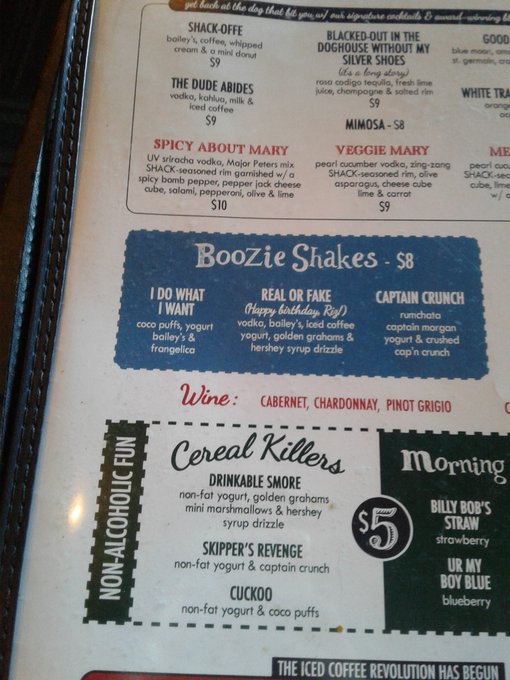The photograph captures a close-up section of a restaurant menu, featuring a white background with a selection of creatively named cocktails and other beverages. The topmost portion of the menu lists the cocktails in bold black lettering:

- Shack Off: Bailey's Coffee Whipped Cream - $9.00
- The Dude Abides: Vodka, Kahlua, Milk, and Nice Coffee - $9.00
- Spicy About Mary: UV Sriracha Vodka - $10.00
- Blacked Out in the Doghouse Without My Silver Shoes - $9.00
- Mimosa - $8.00
- Veggie Mary - $9.00

Below this section is a blue area titled "Boozy Shakes" in white lettering. The menu describes decadent shake options:

- I Do What I Want: Cocoa Puffs, Yogurt, Bailey's, and Frangelico
- Real or Fake: Happy Birthday - Vodka, Bailey's, Iced Coffee, Yogurt, Golden Grahams, and Hershey's Syrup Drizzle
- Captain Crunch: RumChata, Captain Morgan, Yogurt, and Crushed Captain Crunch

Additionally, there is a selection of wines listed:

- Cabernet Sauvignon
- Cabernet Chardonnay
- Pinot Grigio

For non-alcoholic options, the menu offers a variety of fun drinks under "Non-Alcoholic Fun," priced at $5.00:

- Serial Killers
- Drinkable S'more
- Skipper's Revenge
- Cuckoo
- Morning, Billy Bob Straw
- You're My Boy Blue